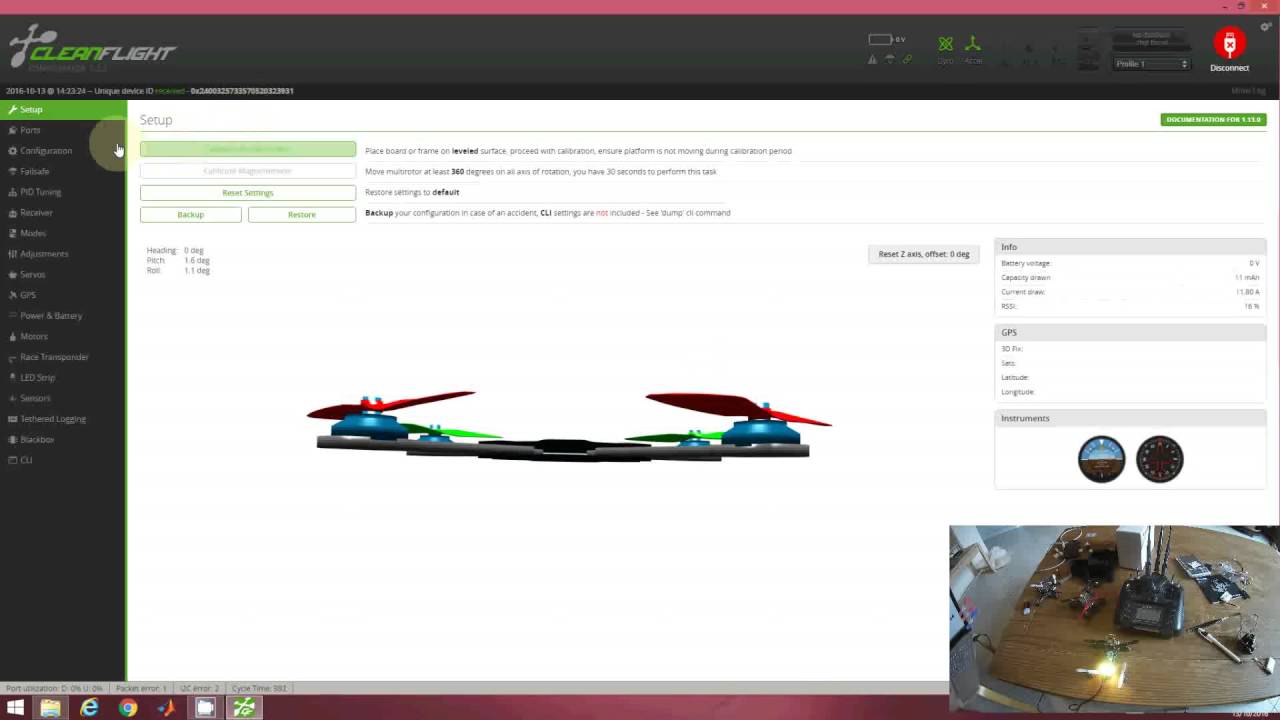The screenshot showcases a webpage interface designed for managing drone settings. At the top, there is a hot pink header featuring two black squares representing minimized windows on the right-hand side. Below this, a dark grey bezel hosts a fidget spinner-like icon, resembling a cross with circular ends, and varying shades of grey. To the right of the icon, the word "CLEAN" is written in bold, green uppercase letters, followed by the grey text "SPLITE".

Adjacent to this section, several icons appear on the right-hand side, including a green pinwheel and a share button composed of a vertical line with two diagonal lines—each ending in a circle—forming a triangular share symbol. Further right, a red circle with a USB-like symbol and a white 'X' inside suggests a disconnected state, substantiated by the white text "DISCONNECT" beneath it.

On the left-hand side, a vertical bezel presents multiple menu options. The currently selected option, "SETUP," is accompanied by a wrench icon and highlighted, while subsequent options are listed in grey text. These include:
1. "PORTS" with a plug icon.
2. "CONFIGURATION" with a gear icon.
3. "FAILSAFE" (the image is slightly blurred).
4. "PID TUNING" with a square and an upward arrow icon.
5. "RECEIVER" with a square icon.
6. "MODES" with two rectangle icons.
7. "ADJUSTMENTS" with vertical lines and intersecting smaller lines.
8. "SERVOS" (possibly) represented by a white box.
9. "GPS" in capital letters.
10. "POWER AND BATTERY" with a battery-like rectangle icon.
11. "MOTORS," although the adjacent icon is unclear.
12. "RACE TRANSMONITOR" with an unreadable icon.
13. "LED SETUP."
14. "SENSORS."
15. "TETHER LOGGING."
16. "BLACKBOX."
17. "CU," associated with a square icon.

Centered in the content area is a mockup of a drone. This drone features cylindrical components in teal, with red blades at the front and lime green blades at the rear, all attached to a dark grey body.